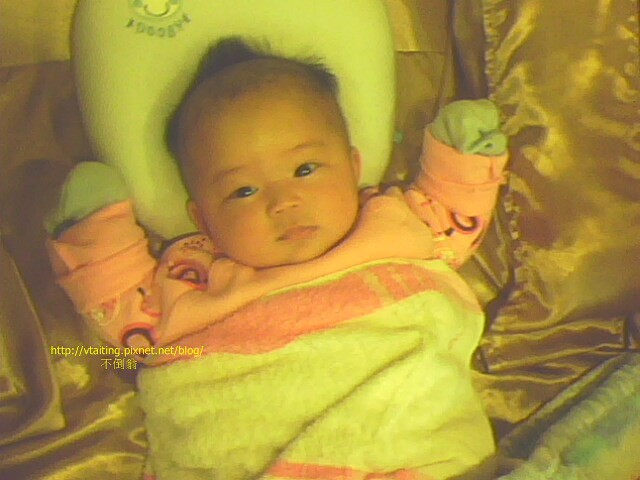The image depicts an adorable Asian baby, centrally positioned, with their head gently resting on a white pillow. The baby is looking directly at the camera, showcasing their cute button nose, dark eyes, and a tuft of black hair standing up. They're bundled up in a pink sweater that covers them completely, including their hands, which are either green or blue mittens. The baby is wrapped in a multi-colored blanket featuring shades of yellow and pink, and some green. The baby appears to be laying on a bed adorned with satin sheets and surrounded by fabric in various colors like yellow, green, pink, and gold. The photo has a yellowish tint, making it difficult to discern if it’s an old photograph or affected by poor lighting. Additionally, there is a web address, http://vtaiting.picsnet.com, accompanied by some Chinese text towards the bottom left corner of the image. The setting seems to be indoors, but the exact time of day is unclear. The warm and cozy arrangement enhances the baby's cherubic charm.